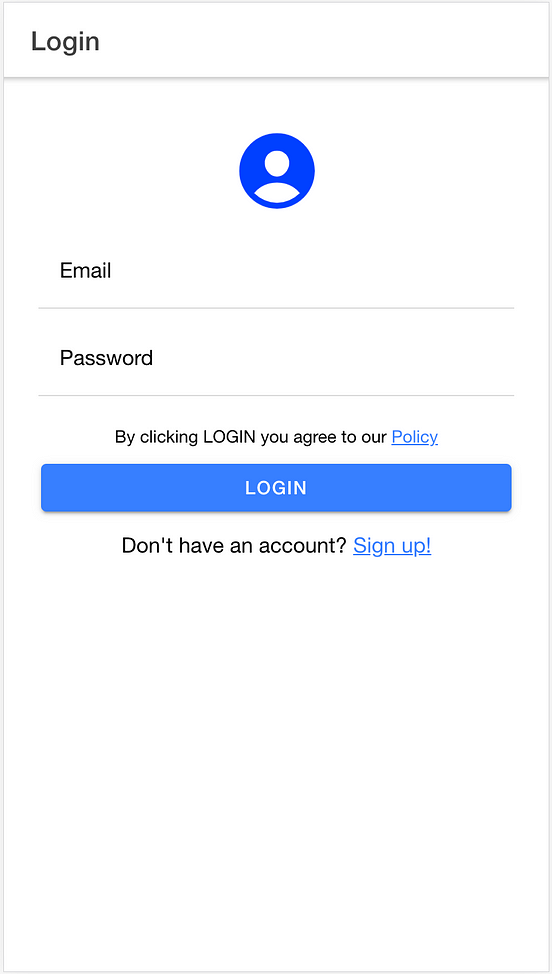This vertical screenshot features a straightforward login page with a minimalist design and a thin gray border framing the entire image. At the top, a thin gray horizontal line separates the header area, where "Login" is displayed in black text in the upper left corner. Below the header, a large, bright blue circle takes center stage, containing an icon of a profile picture—depicted as a white silhouette of a face and torso against the blue background, indicating that no profile picture has been added.

Following this, the form elements are arranged in a clean, linear fashion. "Email" is indicated on the left side, underneath which runs another thin gray line. "Password" follows in a similar manner, with its own separating line beneath it. Just below these fields, centered text in a smaller font reads, "By clicking Login, you agree to our Policy," with "Policy" highlighted in blue and underlined, suggesting a hyperlink.

The main actionable element, a long blue login button, is prominently placed next. The word "Login" is centered on the button in white text, making it highly visible and inviting. Below this button, another centered text line reads, "Don't have an account? Sign up," with "Sign up" underlined and highlighted in blue, encouraging new users to register.

The bottom portion of the image is left intentionally blank with white space, enhancing the clean and uncluttered appearance of the login page.